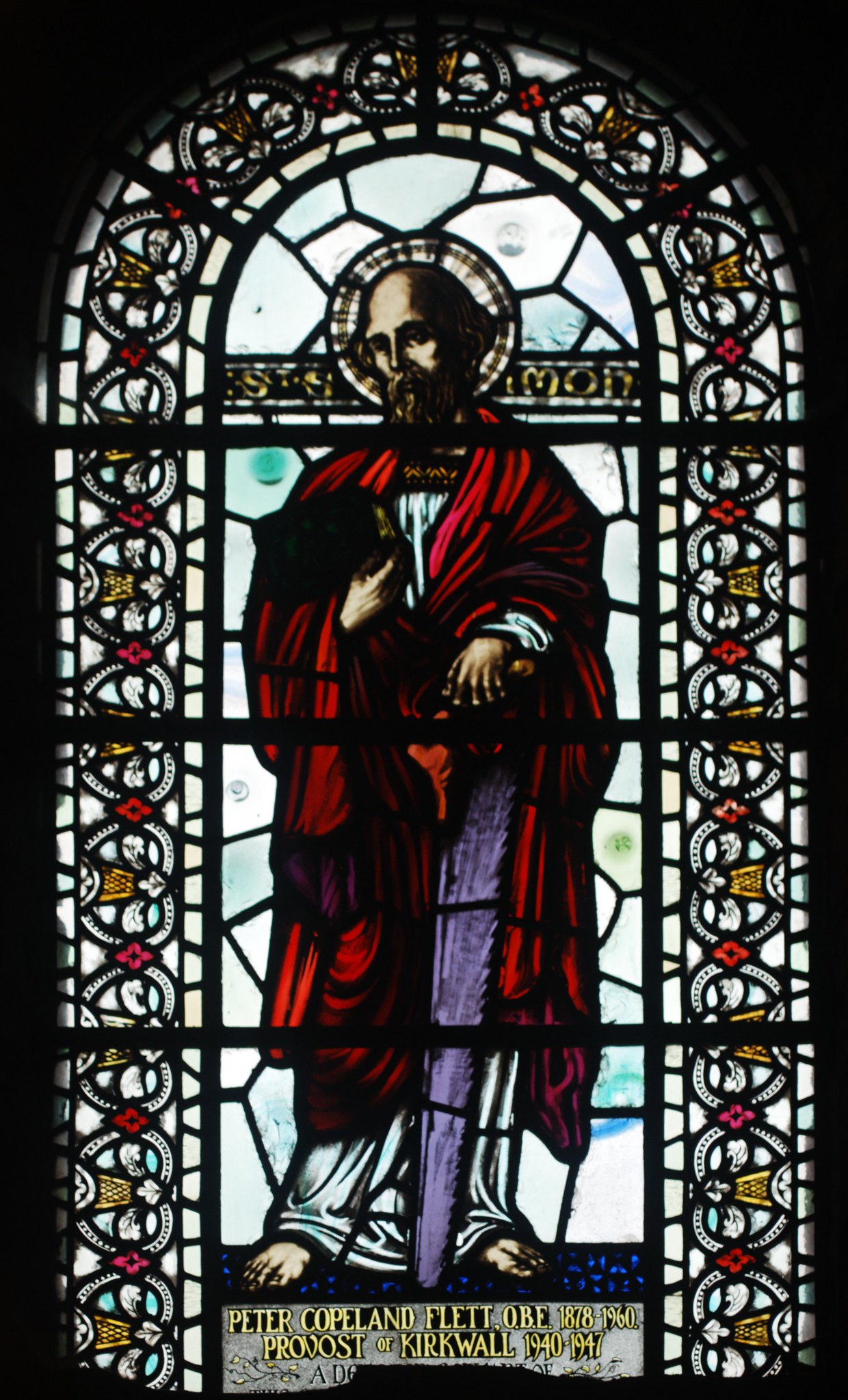The image depicts a large, ornate stained glass window, likely situated in a church. The window is comprised of four panels: three rectangular ones aligned horizontally, capped by a half-circle panel at the top. Surrounding the edges is a decorative border featuring alternating blues, golds, whites, and red flowers between each symbol. 

At the center of the window is a barefoot man with a halo, suggesting he is a holy figure or a saint. He wears a rich scarlet red cloak over a white gown, complemented by a purple sash. His bald head is bowed slightly, and he holds a book in his right hand. Intricate colors such as white, pale blue, ocean blue, yellow, black, and purple enhance the detailed setting.

Beneath this figure, inscribed in gold writing, are the words: "Peter Copeland Flett OBE 1878-1960, Provost of Kirkwall 1940-1947." This inscription likely honors the individual portrayed in the stained glass, cementing his significance to the location.